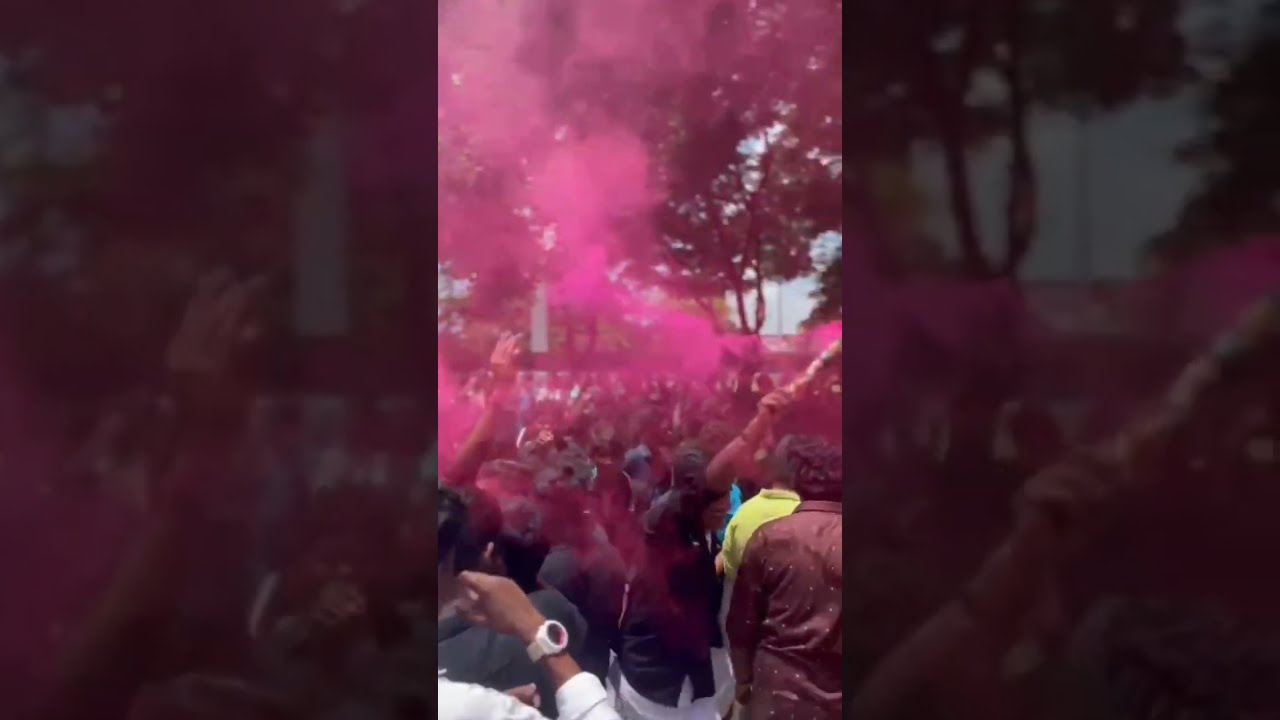In the center portion of this triptych image, enveloped by darker, less discernible left and right sections, a hazy scene unfolds with dense pink smoke filling the air. The vibrant smoke is emitted from smoke sticks held aloft by participants in what could be a protest, demonstration, or public gathering. The crowd, largely turned away from the viewer, obscures their identities. Notably, one individual near the bottom-left wears a white shirt and a prominently thick white-banded watch, extending their hand forward. Nearby, another figure in a bright yellow shirt stands out, as well as a person to the lower right clad in a light maroon-brown coat. Amidst the pink haze, a person is distinguishable holding a raised stick emanating the smoke. Background details feature looming deciduous trees with green foliage under a hazy sky, adding to the scene's atmospheric tension. The cumulative visual is set within three sections, with the outer parts being darker and more abstract, framing the central image.